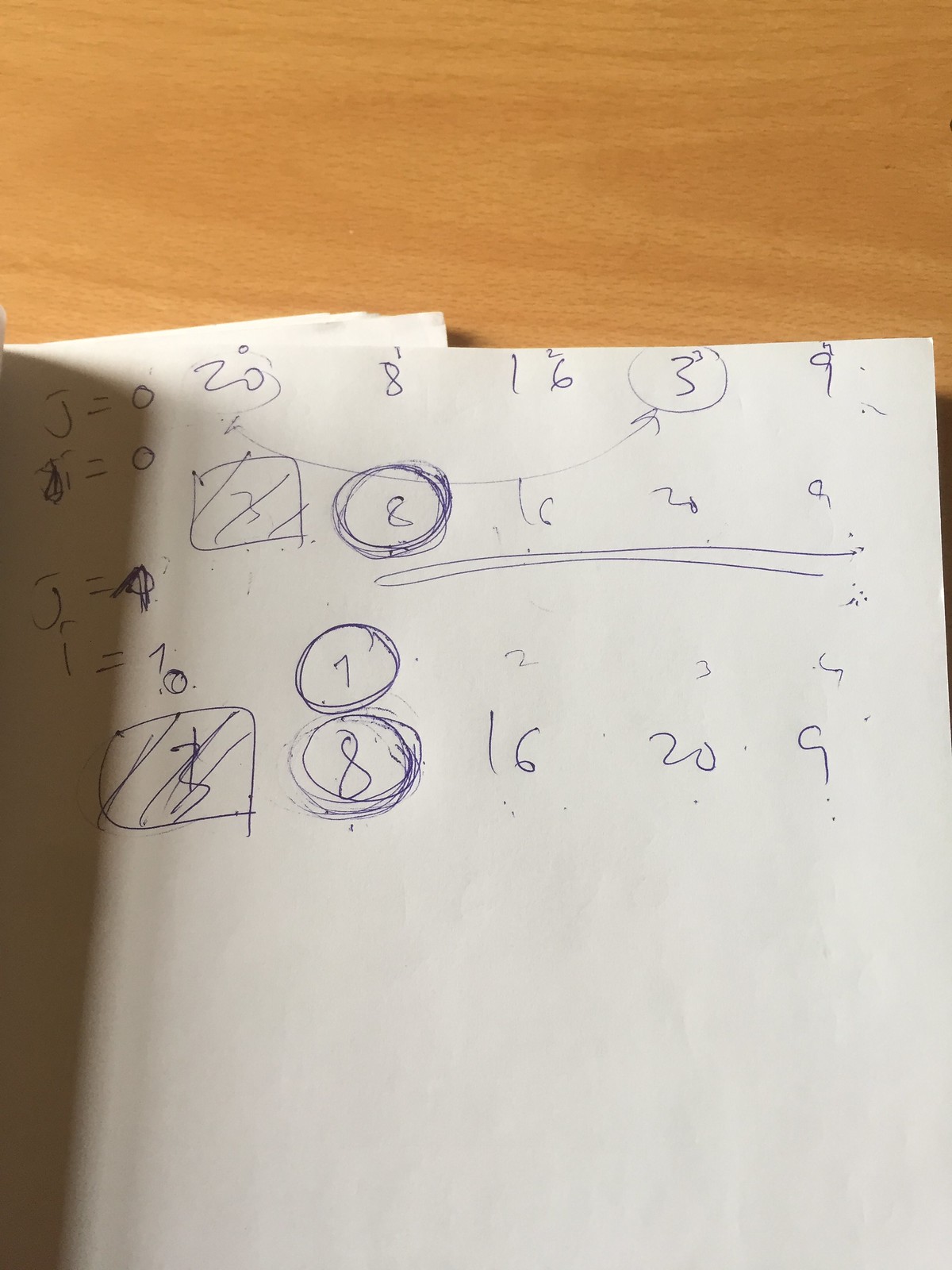A collection of white sheets of paper rests on a slightly dark pine wood surface, prominently displaying its rich brown grain lines. The papers, seemingly used as scratch paper for solving arithmetic or algebraic problems, are filled with a multitude of numbers and letters written in blue ink. At the top left of the paper, the first row of text begins with "J = 0, 20, 8, 16, 3, 9." In addition, a square with the number "3," which has been scratched out, is visibly present, hinting at a correction or change in the calculations. The scene captures a moment of mathematical problem-solving in progress against the rustic background of the wooden table.